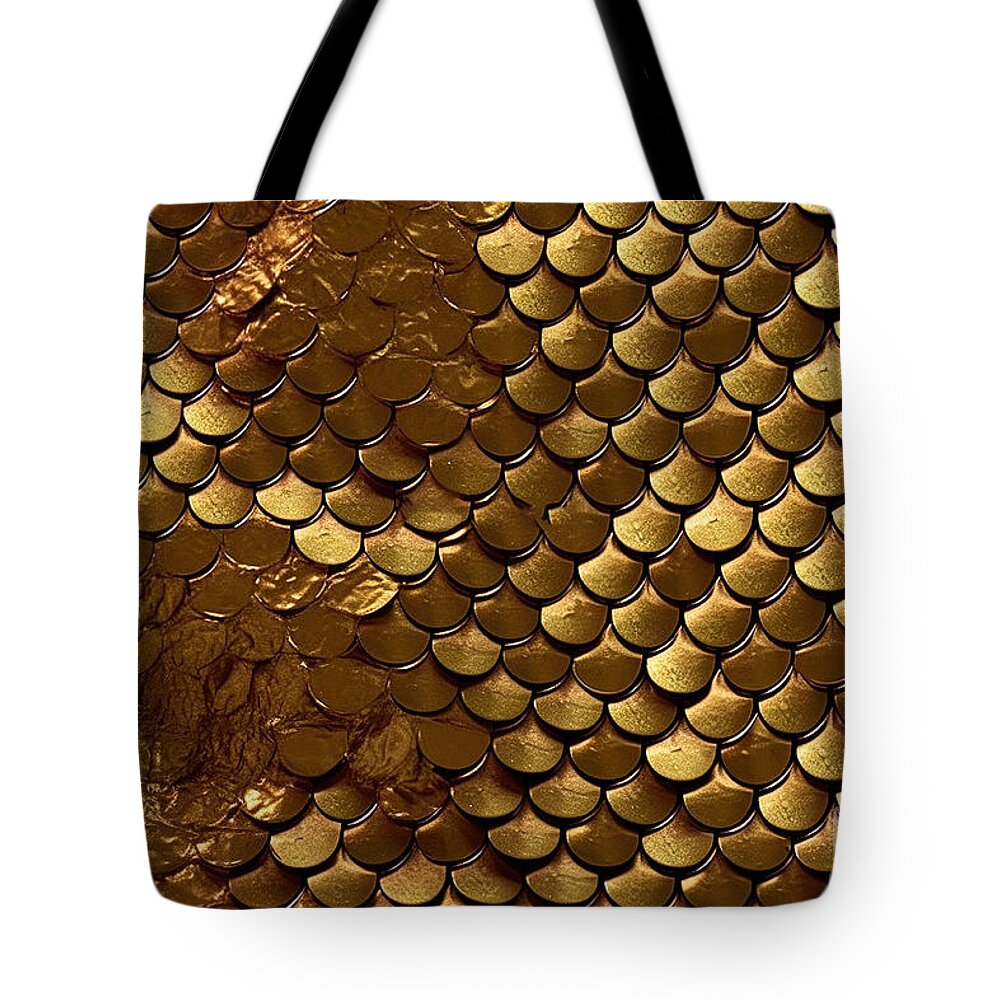The image depicts a square handbag set against a completely white background. The handbag features a striking design that resembles fish or snake scales, with an intricate pattern of alternating golden, brown, and dark golden hues. The scales appear near perfect on the right side, though they become slightly smeared and less defined on the left and the top. The bag is equipped with black handles that partially extend out of the image, hinting at its functionality as a purse or handbag. With no other items present in the image to provide a sense of scale or context, the focal point remains on the handbag's ornate, scale-like exterior.